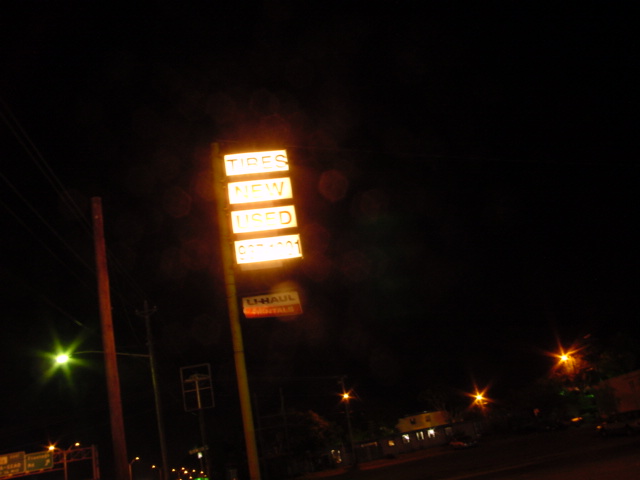The image captures a nighttime cityscape featuring a series of lit-up, rectangular signs stacked vertically on a long metal pole. The top sign glows with the word "TIRES" in black text, followed by "NEW" and "USED" below it, while the fourth sign is unreadable due to glare. Under these illuminated signs, a smaller, non-lit sign reads "YOU HAULT" in black text. To the right of the pole, there is a building with illuminated entrances, adding a warm glow to the scene. The left side of the image reveals several street lights emitting green and yellow hues, along with street signs and other poles, including one with a reddish-brown color. The image is dominated by a vast, black night sky that forms the backdrop for this urban setting, with various light sources creating an interplay of glares and reflections.